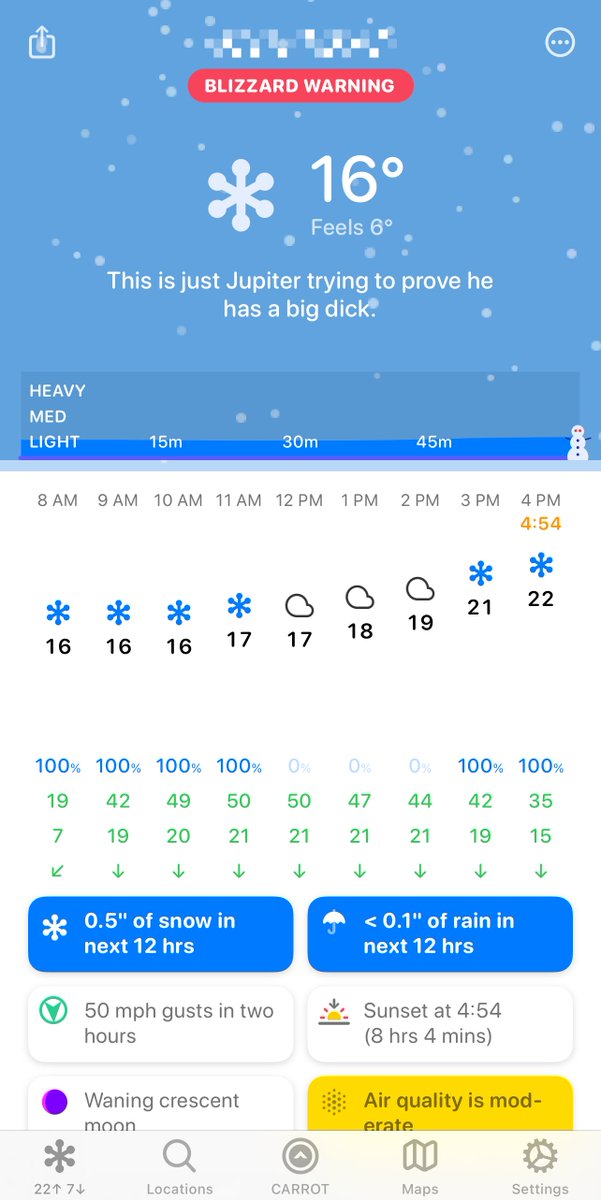The image is a screenshot with a light blue background and white text, illustrating a weather alert. In the upper-left corner, there is a share button, and in the upper-right corner, a menu icon. Snowflakes are depicted falling throughout the background. Prominently at the top of the screenshot, a red warning banner with white text reads, "Blizzard Warning," accompanied by an icon of a white snowflake.

Beneath the warning, bold white text indicates the temperature: "16 degrees, feels like 6 degrees." A humorous and irrelevant comment follows, jokingly stating, "This is just Jupiter trying to prove he has a big dick."

Further down, a white screen displays an hourly forecast from 8 a.m. to 4 p.m., showing the snow probabilities at each hour. The forecast details:
- 8 a.m. - 100% chance
- 9 a.m. - 100% chance
- 10 a.m. - 49% chance

Below the forecast, a blue button reads, "0.5 inches of snow in the next 12 hours." At the bottom of the screenshot, there is a white square indicating that gusts of wind up to 50 miles per hour are expected in the next two hours.